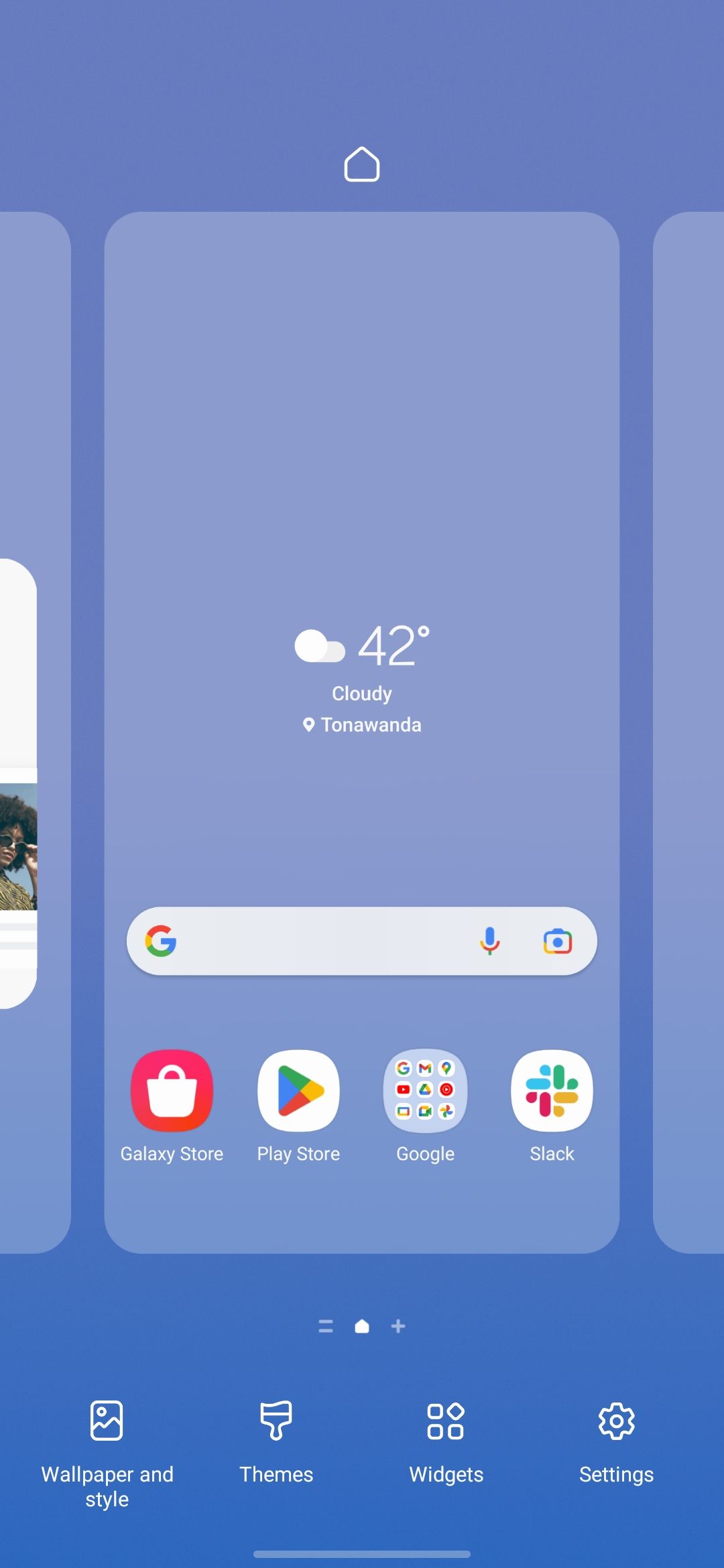This image features a vibrant blue background with a central white outline of a house, suggesting a home screen interface. Positioned around this outline are three rounded squares, each partially cut off at the edges. A slight portion of a white box is visible on the left, but its contents are unclear. On the right, a lighter grayish-blue section appears, displaying a white cloud icon indicating "42 degrees, cloudy, Tonawanda," denoting weather information for a location in Buffalo.

Beneath this is a gray circle featuring the Google logo to the left and a blue circle with a red microphone icon to the right, likely representing voice search functionality. Further below, a horizontal array of icons is spread from left to right:

1. A red circle with a white basket icon, labeled "Galaxy Store."
2. A colorful triangle in blue, orange, and yellow within a white circle, labeled "Play Store."
3. A "Google" icon composed of nine tiny images against a gray background.
4. A white circle with blue, green, and red stubs, labeled "Slack."

Below this row is a darker blue background featuring white font labels and icons in a vertical list:
- "Wallpaper and style" icon depicting a box with a dot, sun, and mountain.
- "Themes" icon represented by a white paintbrush drawing.
- "Widgets" icon showing three squares and a fourth square at an angle.
- "Settings" icon with a gear symbol and the corresponding text.

A gray line marks the lower boundary of the image, centrally aligned at the bottom.